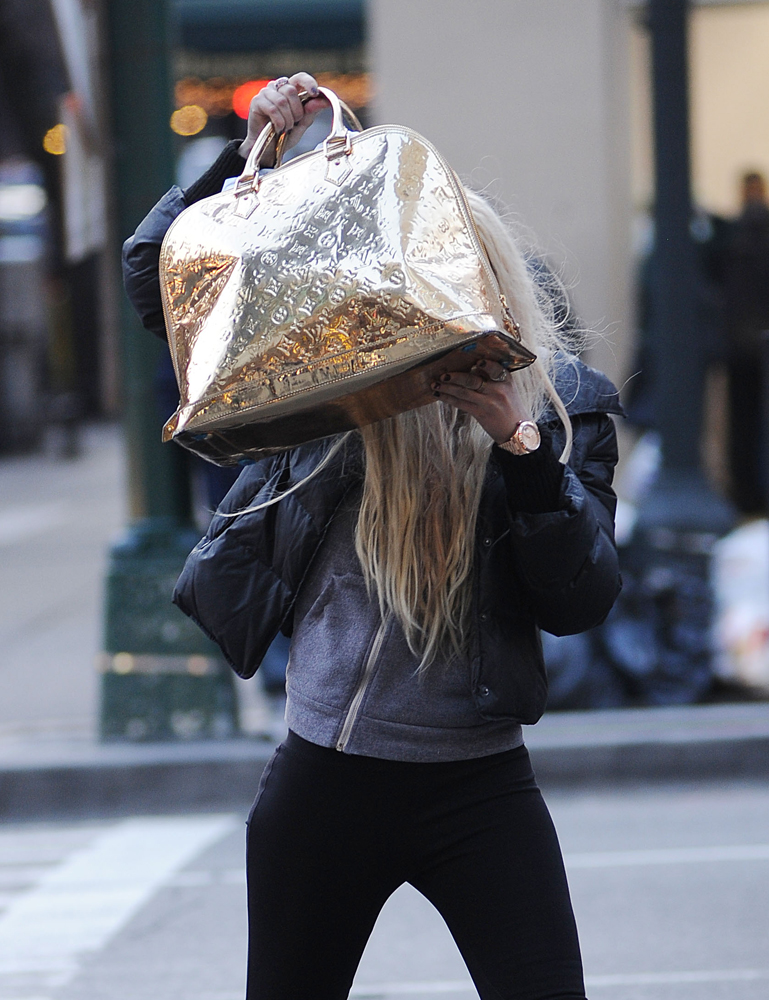In the photograph, a blonde woman with long hair is standing outdoors on a city street, surrounded by blurred elements such as streets, sidewalks, lampposts, a light signal showing a red light, and trash bags across the street. She is dressed in a light gray jumper beneath a poofy dark blue winter jacket and tight black trousers. She wears a gold watch on her left wrist and features several rings on her left hand, specifically on her index and middle fingers. Her nails are adorned with red nail polish. 

The woman is holding a large, shiny golden bag, reminiscent of a bowling bag with gold handles. This bag, possibly made from leather and embossed with symbols or letters, is held directly in front of her face, obscuring it entirely as if she is deliberately trying to hide her identity.